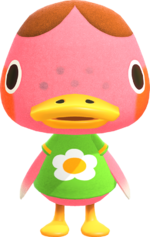This image showcases a highly detailed, contemporary 3D model of a whimsical pink duck, resembling a character from the video game Animal Crossing. The duck is depicted in a childlike, animated style with a bipedal stance. Its round black eyes, accented with a white trim, are set wide apart on its head. The duck has a cute, perm-like hairstyle consisting of two brown circles atop its head, and sports a red blush on its cheeks, adding to its charm. 

It dons a lime green shirt adorned with a white-petaled flower with a yellow center. You can also see the pink belly exposed below this shirt. The duck has a vibrant yellow beak and tiny yellow feet, which are not webbed but resemble duck feet. Additionally, the ends of its wings feature a white tint. The entire character model is set against a plain white background, as if it’s a game asset designed for a digital environment.